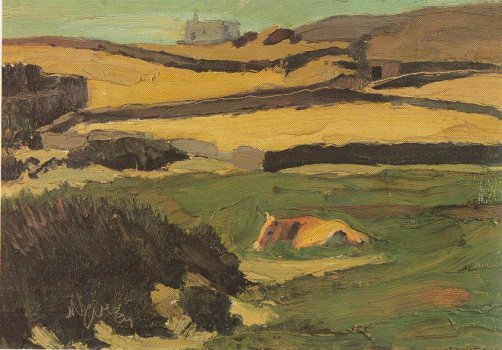In this stylized, post-impressionist nature scene, a vibrant yet indistinct landscape unfolds. The foreground is dominated by rich, almost chaotic greenery that suggests a pasture or grassy field, where the central figure, a cow, rests partially obscured by the tall grass. The details of the animal are pronounced in contrast to its textural surroundings. Moving into the middle ground, the greenery transitions into a yellowish expanse, possibly representing tilled fields or a sandy area, interspersed with a winding stone fence that adds a structured element to the scene.

As the eye travels further, scattered bushes and darker patches add depth, blending into the distant horizon where a castle or monastery stands as a focal point, surrounded by elaborate stone walls. The sky, painted in a subtle gradient of greenish-yellow, underscores the painting’s ethereal quality. The image captures the viewer's imagination with its blend of natural elements and human architecture, accentuated by the artist's signature in the lower left corner. The overall composition, with its layers of color and texture, reflects a deeply abstracted vision of a pastoral landscape.